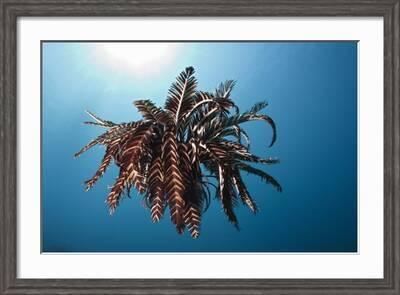This image features a painting in a rectangular, brownish-gray frame with a thin profile. The frame encompasses a white border and a thin black inner line, directing focus to the central artwork. The painting showcases an underwater scene with a predominant blue background and a glow emanating from the top left corner. At the heart of the image is a complex, almost whimsical array of palm tree leaves or feather-like structures that create a circular pattern, which may evoke the appearance of a mythical sea creature or a lionfish. The leaves exhibit an intricate mix of maroon, cream, and brownish-gray hues, appearing wispy and curled, as if gracefully swaying in the water.